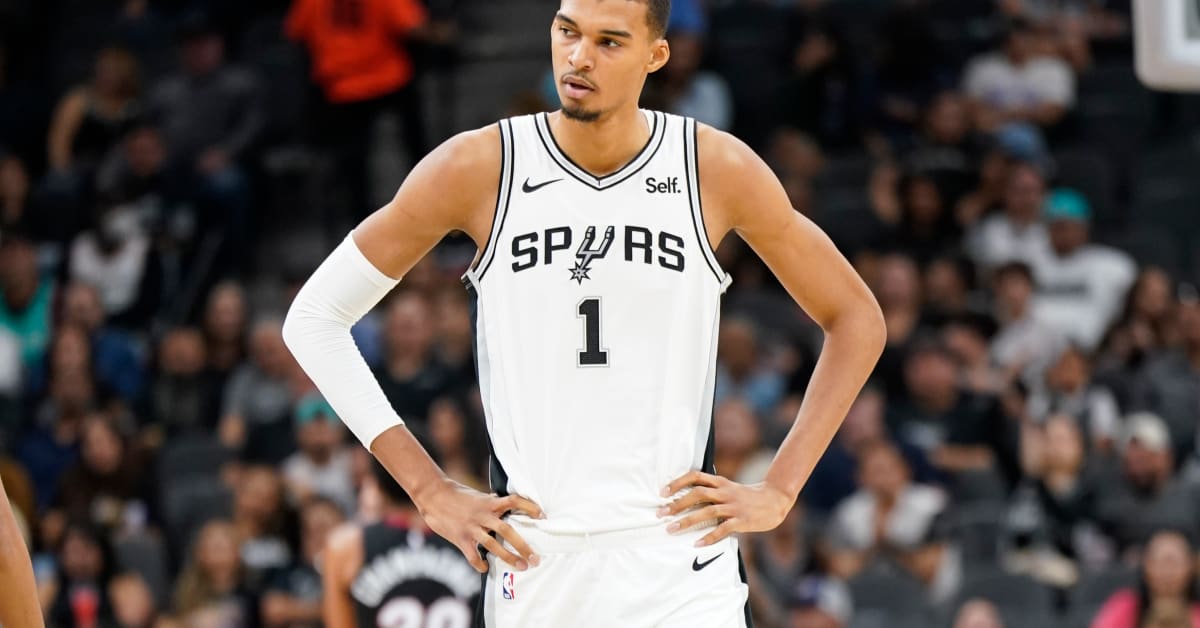The rectangular image prominently features an NBA player from the San Antonio Spurs, wearing the number one jersey. The player, a tall Black male with a short haircut and a goatee, dominates the center of the photograph. He is clad in a white home uniform with black trim, including a white compression sleeve on his right arm. The jersey displays the Nike logo on the top right and the Spurs logo across the chest, with "SELF" as an advertisement on the top left. His white shorts mirror the top with a Nike logo and an NBA logo on the left side. The player is captured with his hands on his hips, a frustrated expression on his face as he looks to his right. Fans in the background, although blurred, fill the arena with indistinct male and female silhouettes. Another competing player in a darker jersey, likely from an opposing team, stands blurred in the background, adding to the competitive ambiance of the arena.